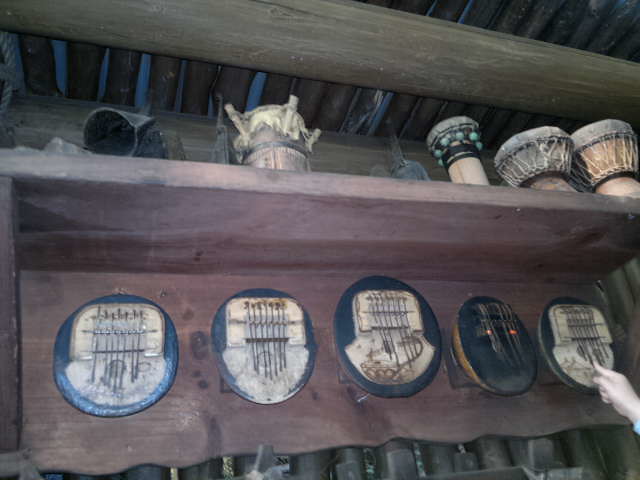The image displays an arrangement of old musical instruments on wooden shelving within what appears to be a warehouse-like space. The wooden shelf, which forms an L-shape with a slab at the back, prominently features several small, decorative drums. There are at least three to four drums, including hand drums and bongo drums. One drum has a white top with tubing extending from the sides, while another, smaller drum is adorned with turquoise and black beadwork. On the underside of the top shelf, there are five circular objects, possibly instruments, resembling drum tops or lids, hanging down. These objects are characterized by a black background with white patches and horizontal metal strips, and they seem to be arranged in a way that might suggest they produce music. Additionally, there is a finger poking at the rightmost circular object, hinting at interactivity.